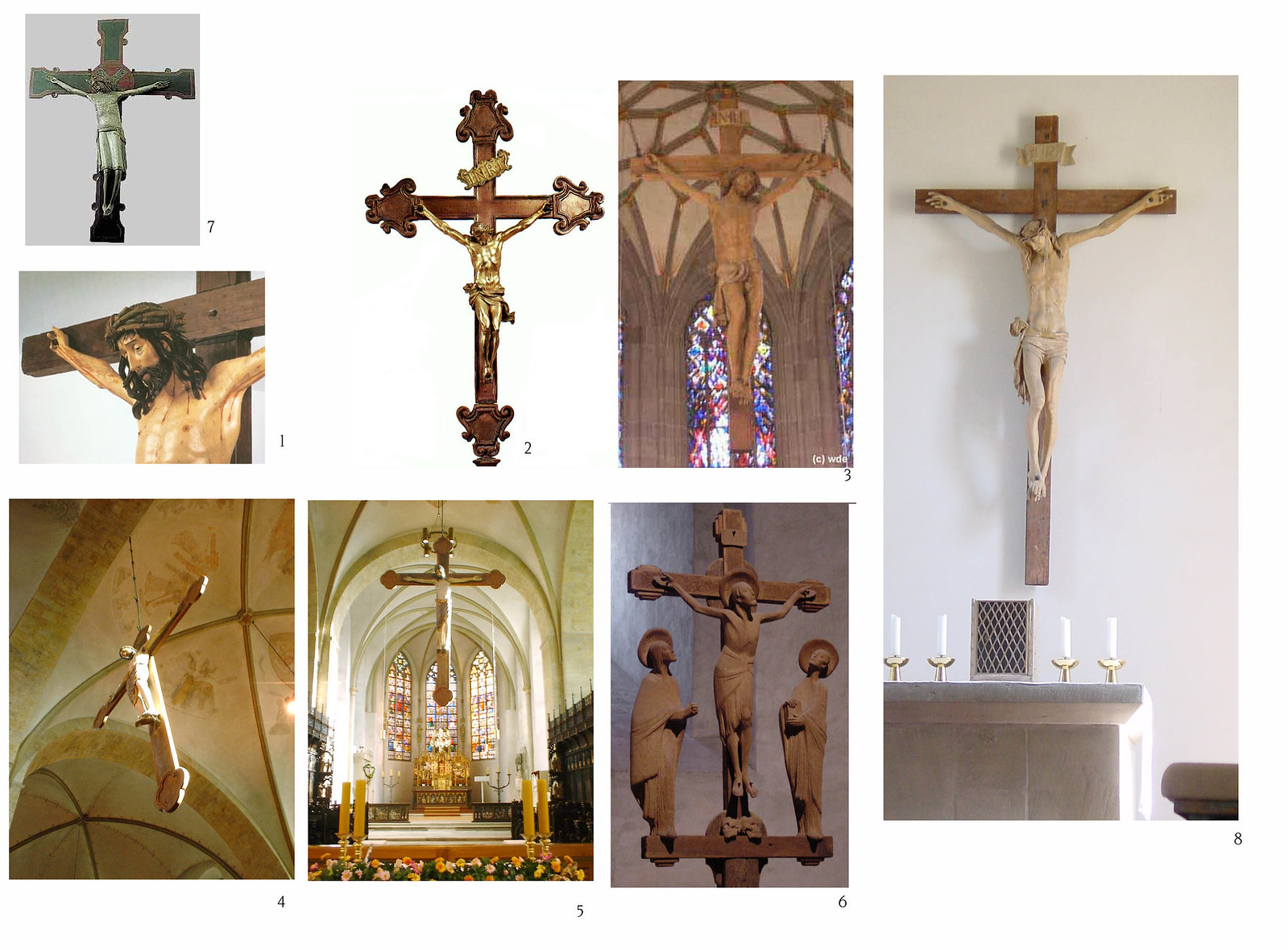This is an intricate photo grid displaying eight distinct images of crucifixes, each numbered from one to eight with a small black numeral. The grid is arranged in a series of rectangular images, with a peculiar layout where the image labeled seven is at the top left, above image one.

1. **Image 7:** Positioned at the top left, it's a small green cross with a light green Jesus figure in front.
2. **Image 1:** A close-up view of Jesus's chest, head, and arms nailed to a brown cross.
3. **Image 2:** Features a gold Jesus statue on a brown cross.
4. **Image 3:** Displays a crucifix hanging inside a tan cathedral, with a light brown Jesus figure visibly suspended in the air.
5. **Image 4:** Shows a brown wooden cross with a brown Jesus figure, set against a tan church ceiling adorned with brown lines, appearing to be suspended from the sky.
6. **Image 5:** Captures an altar where a brown cross with a white Jesus figure is suspended in the air, in a church setting.
7. **Image 6:** Portrays a brown cross with a brown Jesus figure, flanked by two angel statues dressed in white cloaks, both looking up towards the crucifix.
8. **Image 8:** The largest image in the grid, it features a wooden cross nailed to a white wall, with a cream-colored Jesus figure. Below is a white rectangular cabinet or altar with four white candles in gold holders and a rectangular object with a large grated silver screen.

The images are delineated by slight white borders and present various perspectives and environments, including churches and plain backgrounds, highlighting the diverse representations of the crucifix.